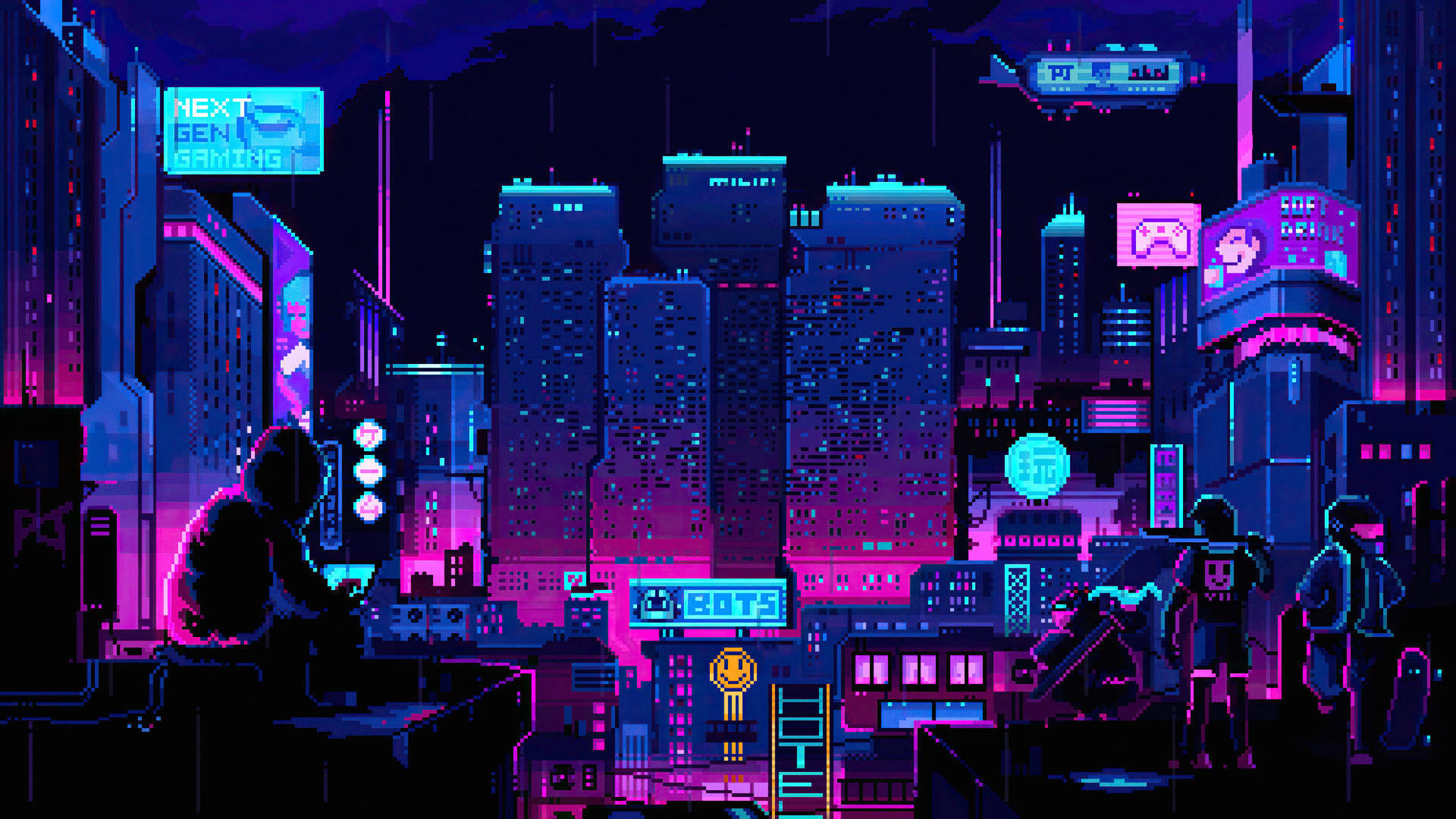The image is a vibrant, pixelated digital depiction of a cityscape, reminiscent of an 8-bit or 16-bit video game design, characterized by neon hues of blue, pink, and purple against a black backdrop. The scene captures an urban downtown area with numerous skyscrapers adorned with illuminated signs and billboards. In the foreground, there are multiple figures: one in a hoodie sitting on a rooftop on the left, and two others on the right, one of whom has a smiley face on the back of their jacket. Prominent signs include "Hotel" in neon green, "Next Gen Gaming," "Soft Drinks," and "Bots" with a smiley face beneath it. The sky above the skyscrapers features what appear to be blue clouds and possibly an airship transporting people, adding to the dynamic and bustling atmosphere of the digital city.